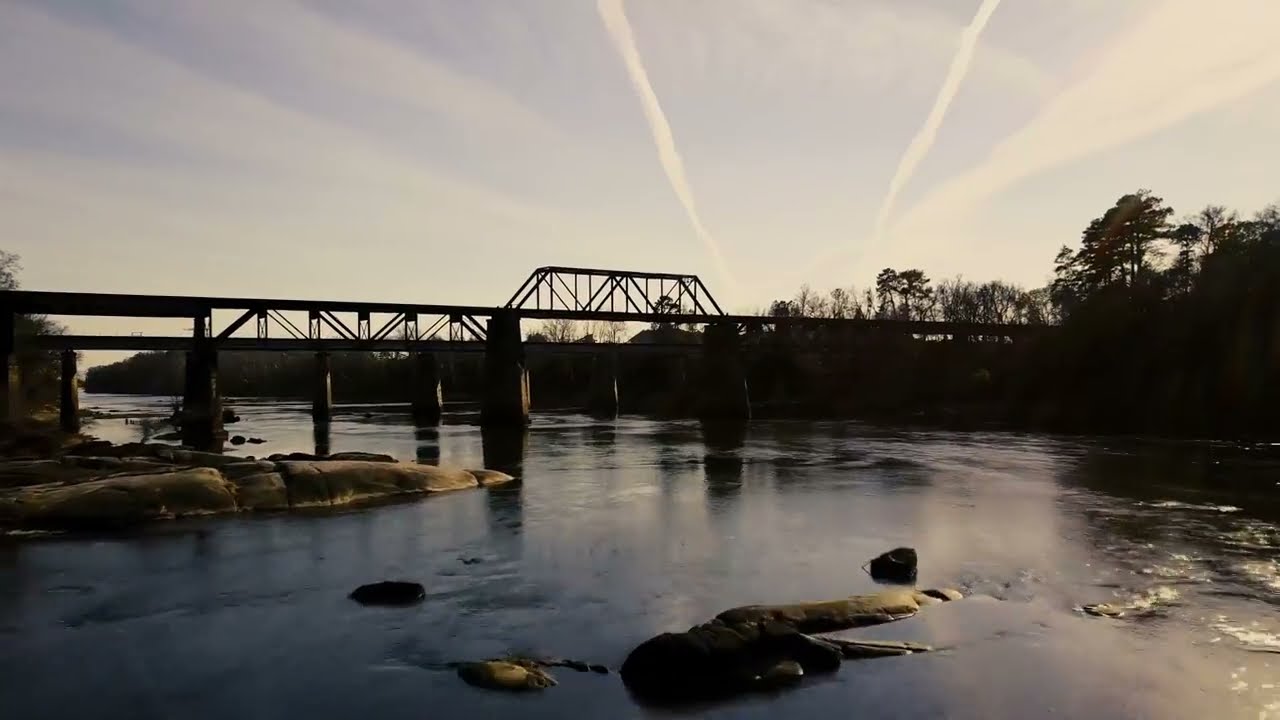This full-color, outdoor photograph, taken during daylight, showcases a serene landscape featuring a narrow metal bridge, likely a train bridge due to the presence of a train trestle, spanning a calm river. The bridge runs horizontally across the image, appearing silhouetted against a backdrop of a blue sky adorned with wispy clouds. The water below is extremely still, with a noticeable current hinted at by the exposed rocks in the foreground. Trees and a forested area frame the scene, providing a lush background. Toward the horizon, a bright light suggests either sunrise or sunset, complemented by two jet streams trailing from an aircraft visible toward this light. The overall scene is devoid of people, boats, or animals, highlighting the tranquility and natural beauty of the setting.